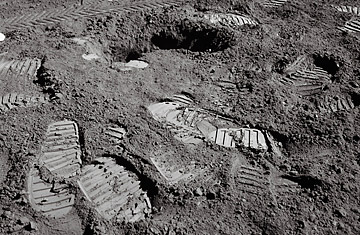This black and white image, measuring approximately 6 1⁄2 inches wide by 4 1⁄2 inches tall, captures the surface of what appears to be the moon, evoking scenes from the historic Apollo missions. Dominating the composition are detailed footprints and tire prints pressed into the fine, clay-like, dusty terrain. Each boot print reveals intricate tread patterns, a testament to the soles designed for the moon's dusty, low-gravity environment. The image, taken in daytime, showcases the imprints in a lighter shade against the otherwise dark, grayish surface. The terrain appears relatively flat, allowing the distinct lines and curves of the prints to stand out. No text or additional elements are present, focusing attention purely on these iconic marks of lunar exploration.